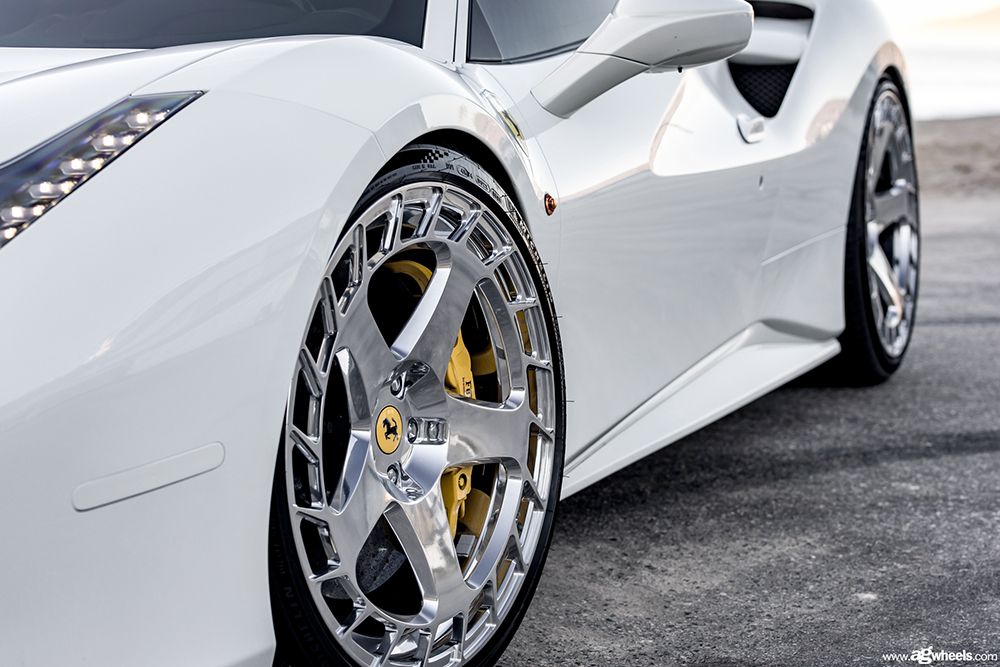This is a close-up photograph of a sleek, high-end, white Ferrari sports car, prominently featuring its left side. The emblems with the prancing horse, set against a yellow background, unmistakably indicate its prestigious Ferrari heritage. The car exudes a sense of speed and luxury, even while stationary. Its sport wheels are equipped with high-performance, thin-sidewall tires, and the disc brakes, visible through the wheels, boast striking yellow calipers. The car has dark, tinted windows and elegant silver hubcaps that add to its high-fashion appeal. Subtle details like the left headlight and side mirror are visible, along with air intakes near the rear wheel. The scene is set outdoors on asphalt under a bright, sunny sky. The car not only looks fast and expensive but also impeccably polished, suggesting it's a new model. The presence of a website, www.agwheels.com, in the bottom right corner hints at a possible focus on custom wheels or automotive accessories.